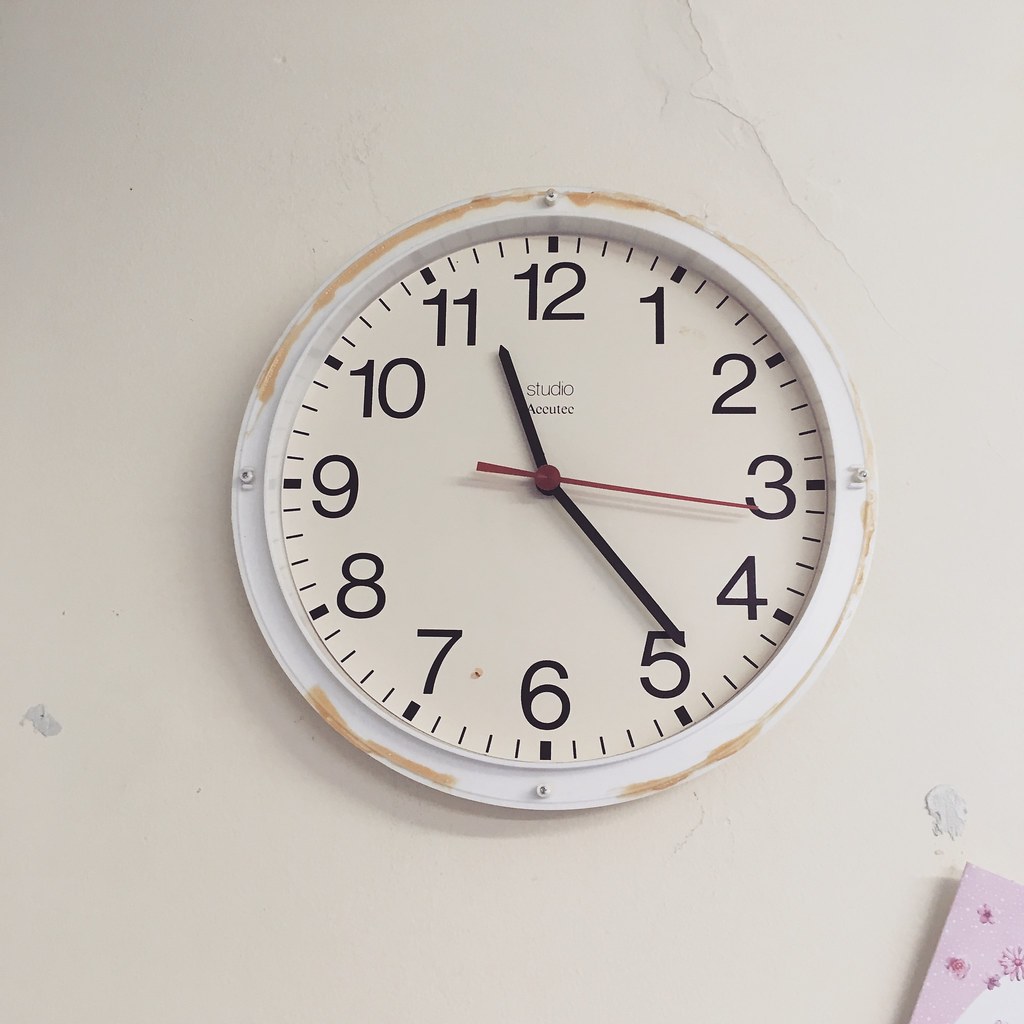This close-up photograph captures a weathered circular clock mounted on a slightly cracked and indented white wall. The clock is predominantly white, though its housing shows patches of light brown where the paint has worn away. Its face, a faded white, is marked with bold black numbers and both dark and thin black hash marks delineating each minute. The branding "STUDIO" and "ACCUTE" is prominently displayed near the center top. The clock's hands are black, with a distinct red second hand; all three are fastened by a small red circle with a black pin. The time displayed is 11:24. Directly below and to the right of the clock, a pink card adorned with hot pink floral designs adds a splash of color to the scene. Additionally, a white, partially cut-off oval shape is visible, contributing to the image's detail.